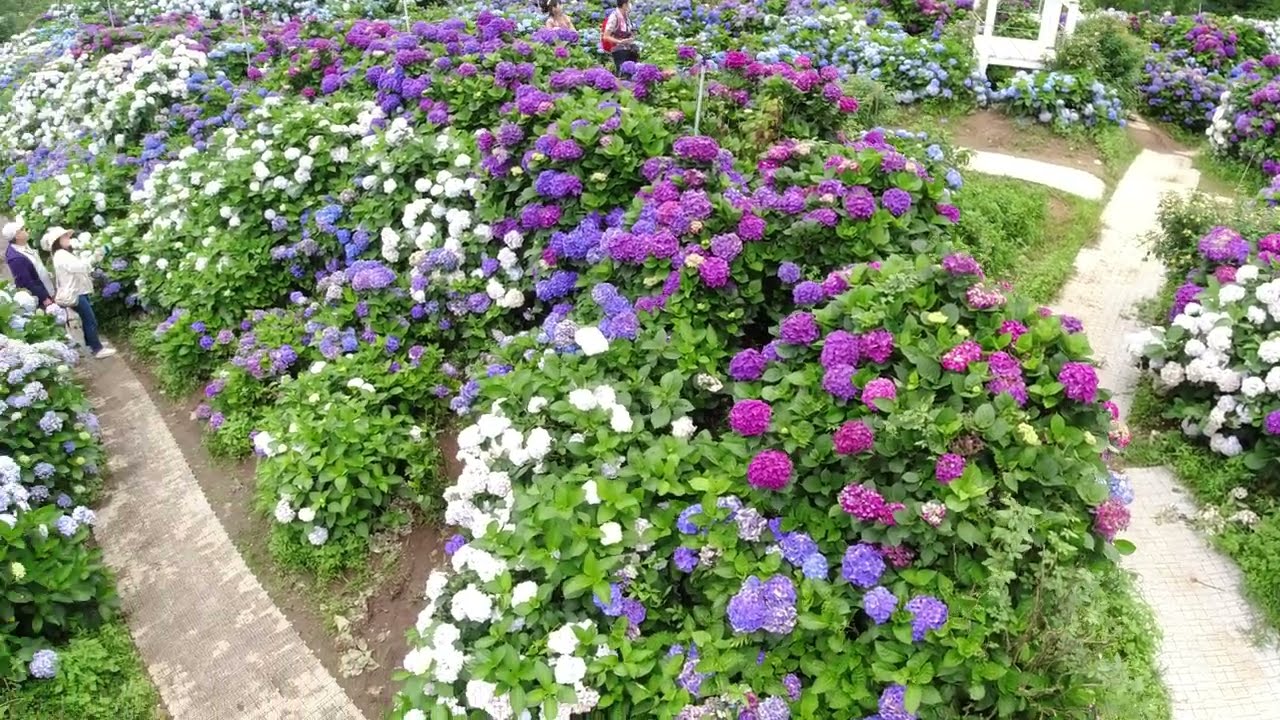This rectangular photograph, taken from an aerial perspective, captures a vibrant garden area dominated by interlocking gray stone pathways that weave through lush green bushes. The garden is densely populated with large, fluffy hydrangeas in an array of colors, including blue, purple, hot pink, lighter pink, and white. On the left-hand side of the image, a woman in a white hat, white jacket, blue jeans, and white tennis shoes is seen savoring the fragrance of the flowers. Standing beside her is a man in a white hat, blue jacket, and white shirt. His lower half is concealed by the lush blooms. The pathways, though mostly a gray stone color, show signs of dirt and garden soil. Elsewhere, further into the image, another couple is visible. One person is attired in a red vest over a white shirt, while another figure appears to be clad either in a tank top or a skin-colored shirt. In the background, the garden seems to rise up a gentle hill, and there appears to be either a gazebo or a bench nestled amidst the flowers, adding to the serene ambiance of this idyllic garden scene.